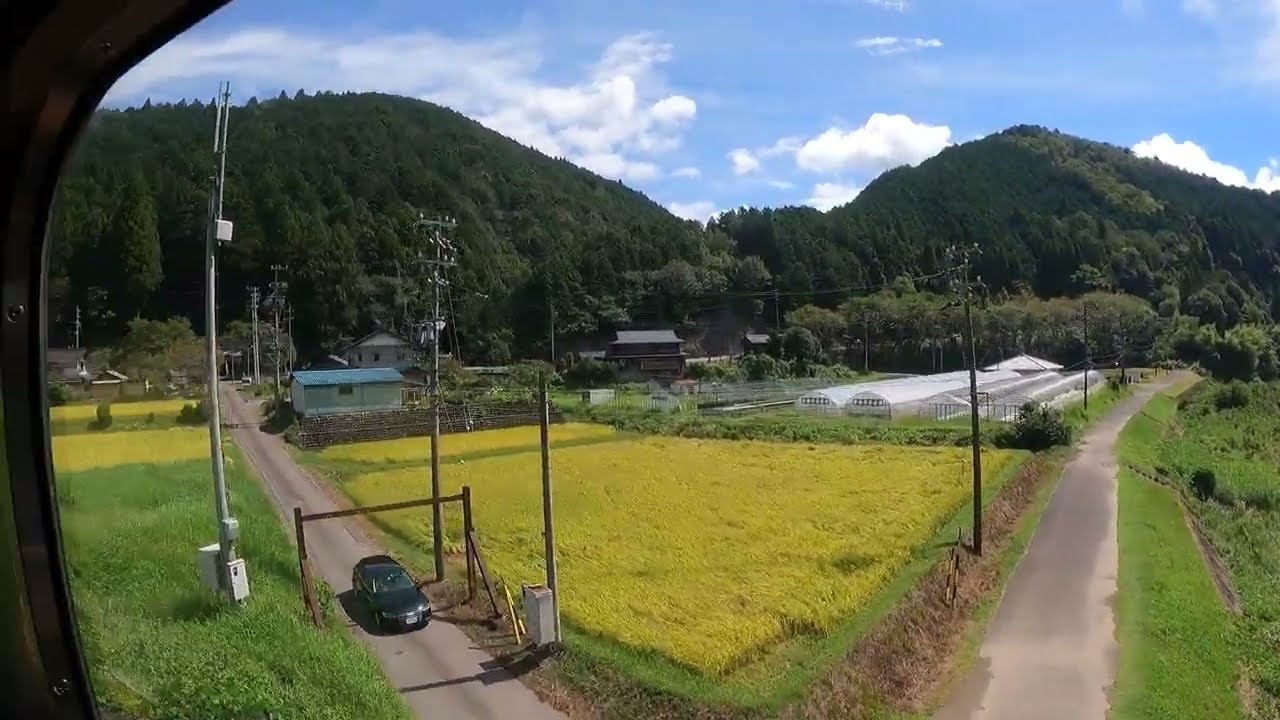This aerial photograph captures a picturesque rural landscape brimming with natural and man-made elements. Taken from a low-flying aircraft, possibly a helicopter, the image is framed from above and brilliantly showcases a vast expanse of fields and pastures intersected by two gray paved one-way roads that fan out from the bottom of the image towards the left and right. A black car is visible traveling along the left road towards the bottom of the scene.

Positioned between the roads is a diamond-shaped patch of land characterized by its light green hue, surrounded by darker green grass. At the far end of this patch, one can see four long, cylindrical white greenhouses lined up in a row. Off to the side of the greenhouses, there are several structures resembling houses, barns, or buildings, complemented by additional infrastructure such as power lines and telephone poles. A drainage canal or irrigation ditch is also visible, designed for managing water runoff.

In the background, the horizon is beautifully punctuated by two imposing, verdant mountains. The taller of the two has a prominent peak that dips down before rising again to the left, creating a dramatic and scenic profile. The landscape looks lush and possibly tropical, suggesting a warm climate reminiscent of regions like California or similar island locales. Above, the sky is a brilliant blue adorned with a few fluffy white clouds, adding to the idyllic and serene atmosphere of this vibrant rural setting.